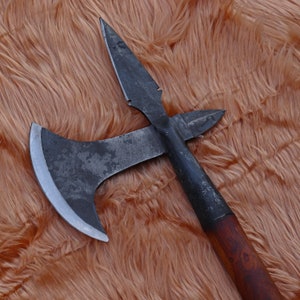This image is a close-up of a metallic weapon, likely an axe with a spear-like pointed end. The main focus is the weapon emerging from the bottom right, showcasing a weathered, dull steel blade and a pointed spearhead. The metal sections appear aged and possibly of historical significance, which could suggest it’s either a genuine artifact or an antique replica. The handle is made of worn brown wood, with visible grain, enhancing its rustic look. A rounded metal piece complements the weapon’s middle section. The entire object rests on a strawberry blonde, long-pile faux fur, which adds a stark contrasting background, resembling soft strands or a hide.